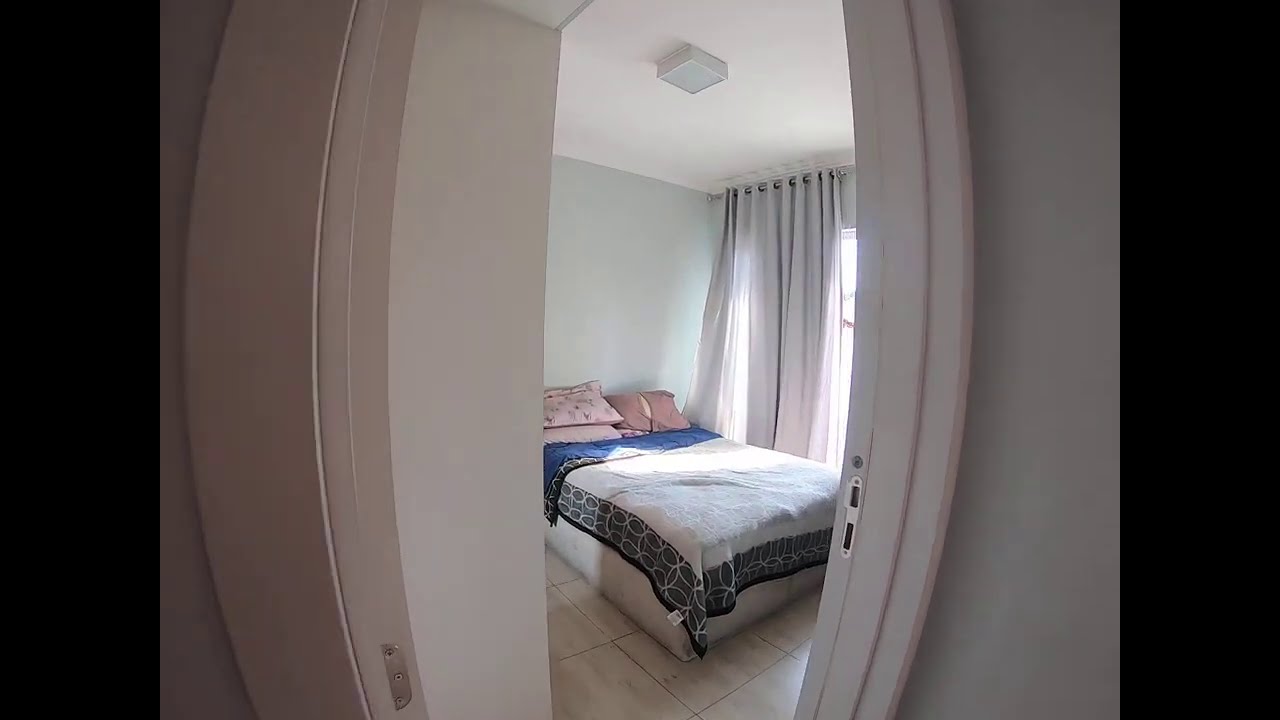This photograph, seemingly taken with a fisheye lens, captures a sparsely decorated bedroom through an open doorway. The walls are a very pale off-white or light tan beige. The floor appears to be tiled in an off-white color matching the walls. The focal point of the room is a bed, which appears to have its mattress and box frame resting directly on the floor. The bed is adorned with a white comforter featuring a red border and circular white designs. The folded sheet near the pillows reveals a blue underside. At the head of the bed are three beige or tan pillows stacked neatly against the wall. To the right, there's a large gray window with a matching floor-to-ceiling curtain that allows daylight to stream in, illuminating the room. A ceiling light fixture, square and box-like, hangs directly above the bed, casting light downwards. The slightly curved doorframe, attributed to the fisheye effect, frames this minimalist and serene space.